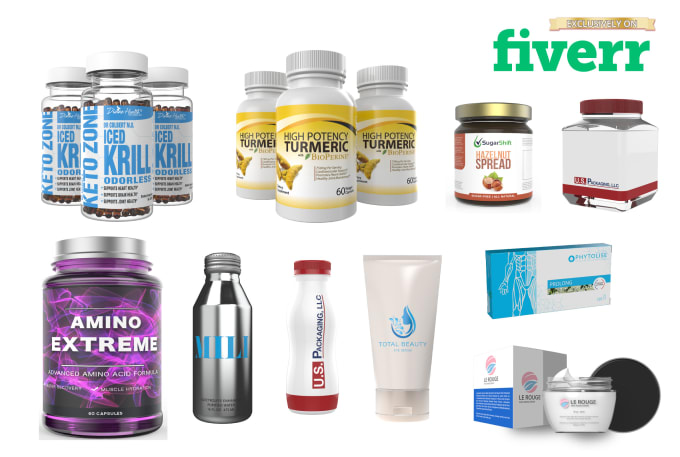In the image, an assortment of health supplements is prominently displayed. The collection includes bottles of krill oil, turmeric, and Amino Extreme, each presented in screw-top containers. The Amino Extreme bottle stands out with its vibrant purple label, while the turmeric supplement features a striking yellow design. Among the assortment, there's also a blue and white packet, which is the most colorful item in the display. Additionally, the scene includes a couple of tubes and a packet, although the exact details on some items are not entirely clear due to small, unreadable text. At the bottom of the image, several face care products are arranged in glass jars with screw tops, one of which has a black lid and is positioned on its side. The overall presentation highlights a variety of health and wellness products.